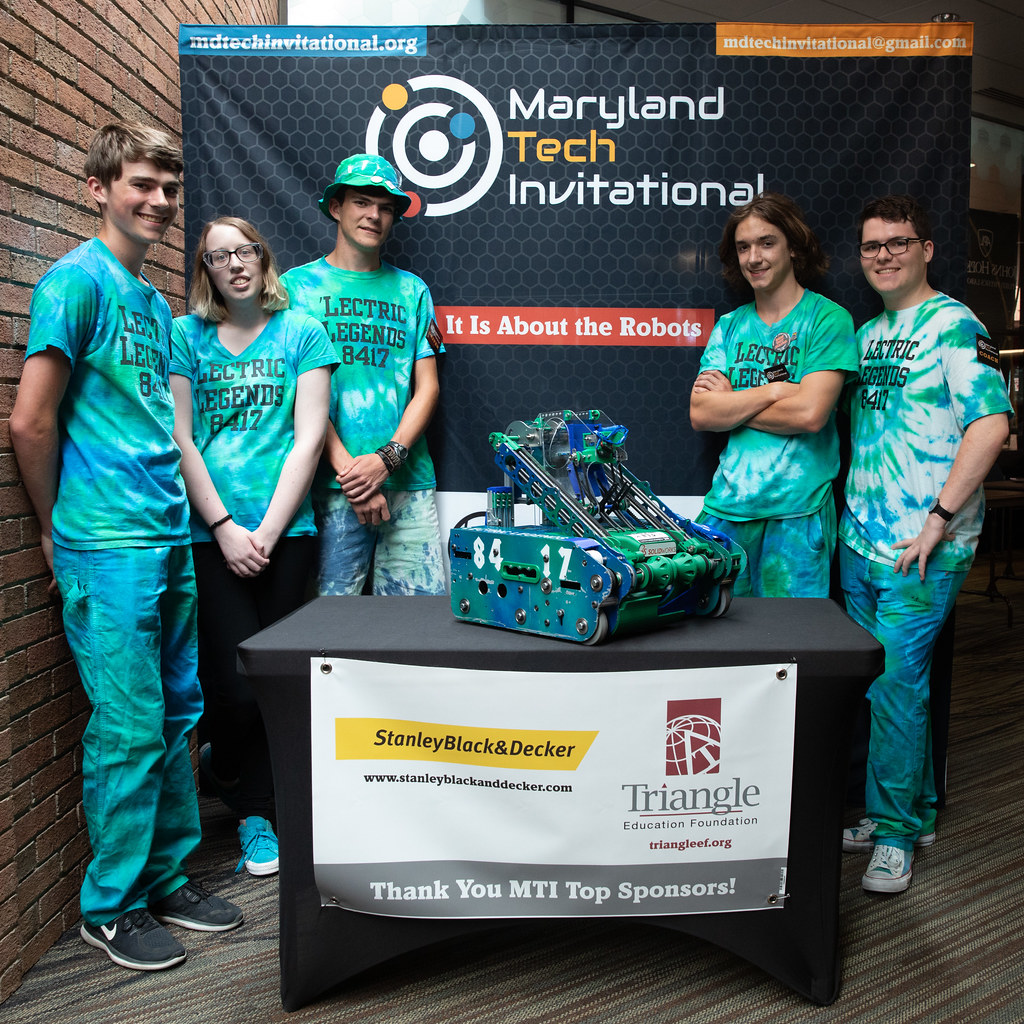In the image, five young college students are gathered around a black table that displays a blue and green robot echoing the tie-dye colors of their shirts and trousers. The students are part of the "Electric Legends 8417" team, showcasing their creation at the Maryland Tech Invitational. Behind them, a detailed stand features a hexagonal honeycomb pattern with text such as “Maryland Tech Invitational” in white and orange, the website “mdtechinvitational.org” in the top left corner, and contact email “mdtechinvitational@gmail.com” in an orange banner in the top right. A red banner across the middle proclaims, “It is about the robots.”

The students are arranged with a young man on the far left leaning against a brick wall, followed by a young woman in glasses with her arms in front of her, a young man in a colorful hat also with his arms in front, another young man with folded arms smiling at the camera, and on the far right, a young man wearing glasses smiling with his hands on his hips. The robot on the table is designed with wheels and a sliding mechanism, mimicking the team’s tie-dye motif. A poster below the table reads, “Stanley Black & Decker, www.stanleyblackanddecker.com, Triangle Education Foundation, triangleef.org. Thank you, MTI, top sponsors."